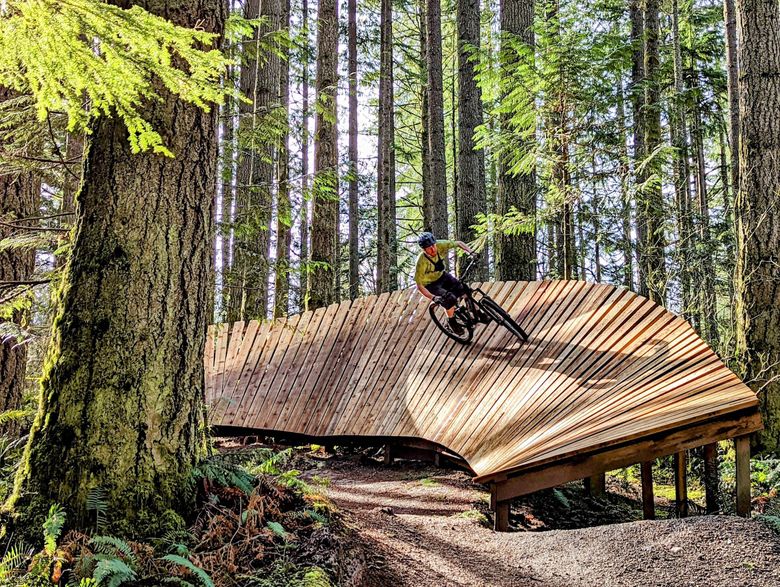In this photograph taken outdoors on a sunny day, a mountain biker is captured in an impressive action shot. The rider, donned in a yellow high-visibility long-sleeve shirt and a blue helmet, navigates a steep, banked curve on a wooden ramp. The ramp, built from many individual wooden planks, is set in a forest, surrounded by tall trees with green foliage and moss. The structure of the ramp is intricate, with boards angled steeply, creating an almost vertical incline in parts, resembling a sideways wooden sidewalk. The scene is likely set in the Pacific Northwest, given the presence of evergreen trees and lush underbrush. As the rider approaches the end of the ramp, which drops off onto a dirt path below, he is angled at about 45 degrees to the ground, indicating significant speed. The background is rich with large trees and ferns, contributing to the natural and rugged atmosphere of the photograph.